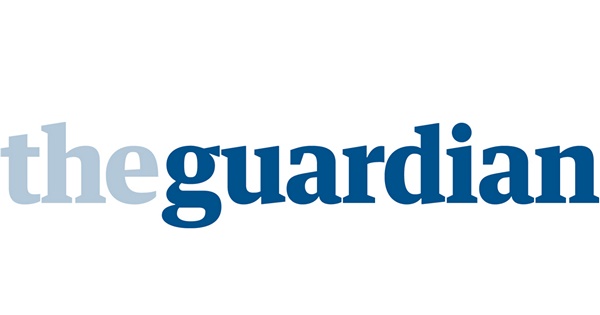The image features the words "theguardian" written as a single continuous string without any space between "the" and "guardian." The text is set against a plain white background without any borders. The word "the" is in lowercase letters, displayed in a pale bluish-gray color, while "guardian" is written in a darker shade, closer to navy blue but not quite as dark. 

The letter "G" in "guardian" is distinctive, resembling an 'O' with a small arrowhead pointing into the right side of the top of the 'O.' Additionally, it features a curly extension that starts from the lower left of the 'O', extends leftward, then sweeps to the right, downwards, back to the left, and finally curls up to join the bottom of the 'G.' 

The dot over the "i" in "guardian" is notable for being a large, filled-in circle. The font resembles a rounded, lowercase version of Times New Roman, with smooth, curved lines rather than angular ones.